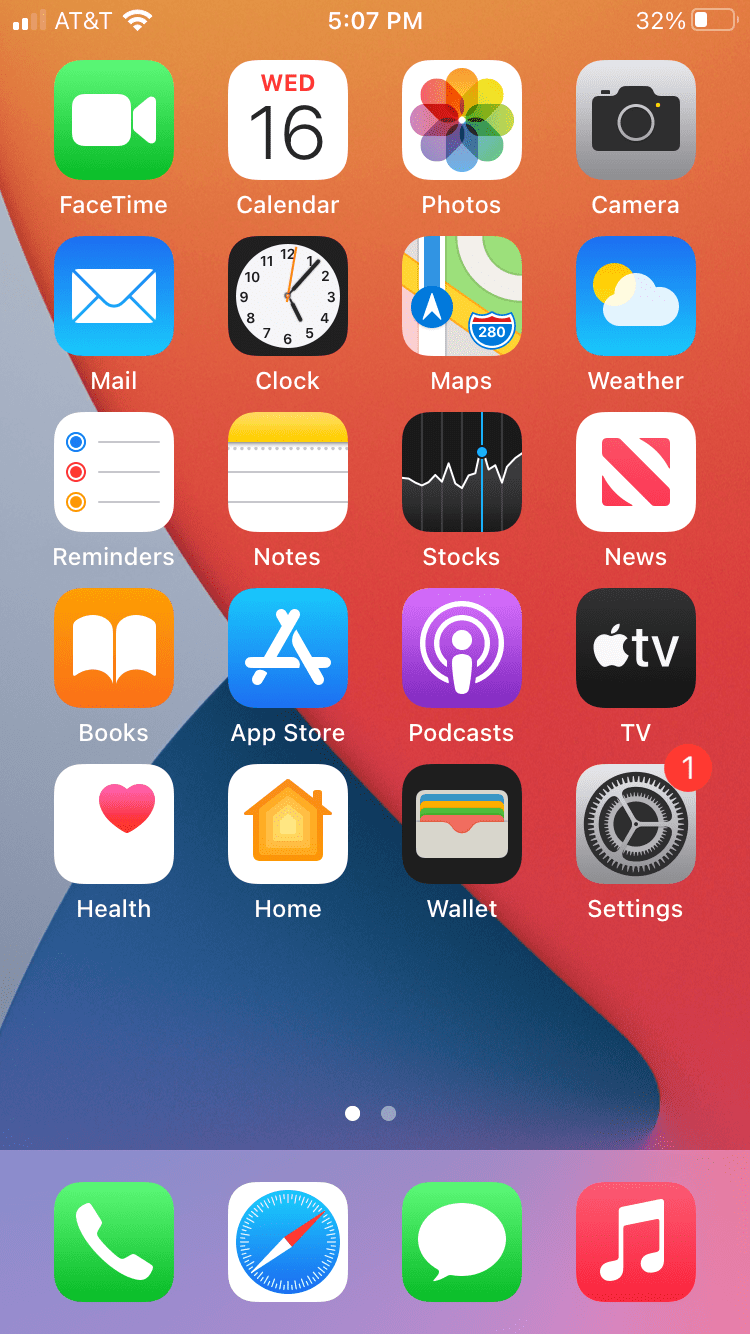This screenshot captures the home screen of a cell phone with a geometric-themed wallpaper. The wallpaper is composed of three distinct color sections: an orange area occupying the upper right-hand side, curving diagonally to the bottom right; a triangular dark blue section at the bottom; and another triangular gray section extending from the lower left corner to the upper right into the center. At the top of the screen are status indicators in white lettering, including two Wi-Fi bars, "AT&T," a Wi-Fi signal, the time "5:07 PM," and a battery icon at 32% with a partially filled white section.

The home screen displays icons organized into columns of four, with four icons per row. The icons have a rounded square shape and white labels. From top left to bottom right, the icons are as follows:

- **First row**: FaceTime, Calendar, Photos, Camera
- **Second row**: Mail, Clock, Maps, Weather
- **Third row**: Reminders, Notes, Stocks, News
- **Fourth row**: Books, App Store, Podcasts, TV (indicating this is an Apple phone due to the presence of Apple TV)
- **Fifth row**: Health, Home, Wallet, Settings

Beneath these icons, there is a filled-in white dot in the bottom center, indicating the current home screen, and a gray dot to the right, denoting additional screens. The bottom banner, which has a grayish-purple-pink hue, features four more icons: a green icon with a white phone receiver (Phone), a blue compass on a white background (Safari), a green icon with a white speech bubble (Messages), and a red icon with white music notes (Music).